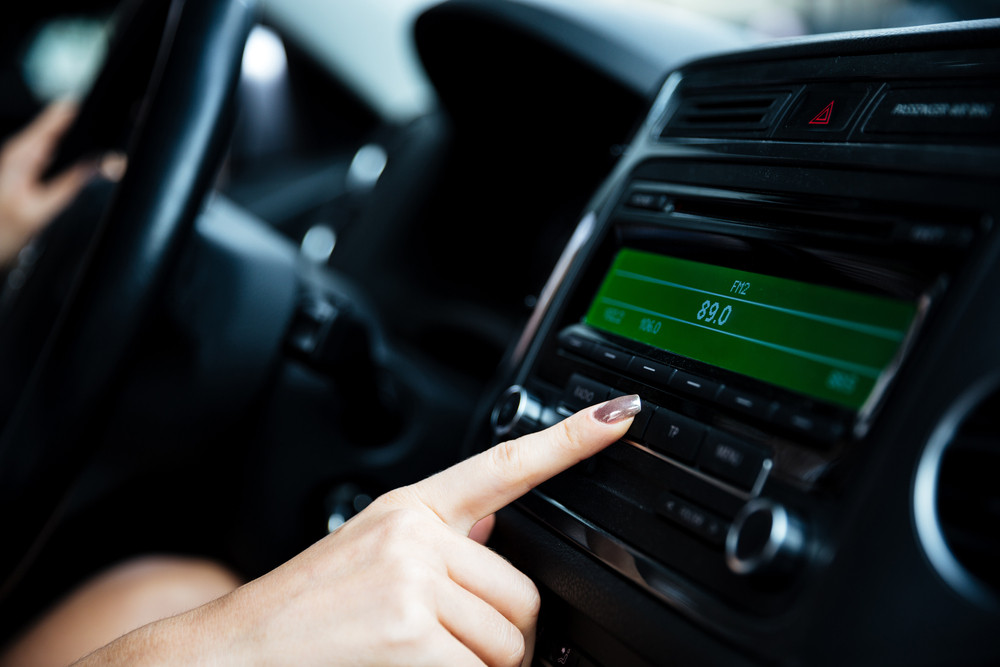In the image, a close-up view of a car's interior is captured with high detail. The focal point is a woman’s right hand, with a well-manicured index finger, pressing a button on the car’s radio console. Her left hand is placed on the black steering wheel, indicating she is ready to drive. The dashboard is adorned with a green digital screen at the top, prominently displaying "FM" and "89.0" on its lines. Below this screen, to the left and right, are numerous knobs and buttons, including one with a glowing orange triangle symbol above it. The interior of the car predominantly features a black finish, and while the image is somewhat blurry, the essential elements are discernible. Additionally, the radio appears slightly older and even includes a CD player component.